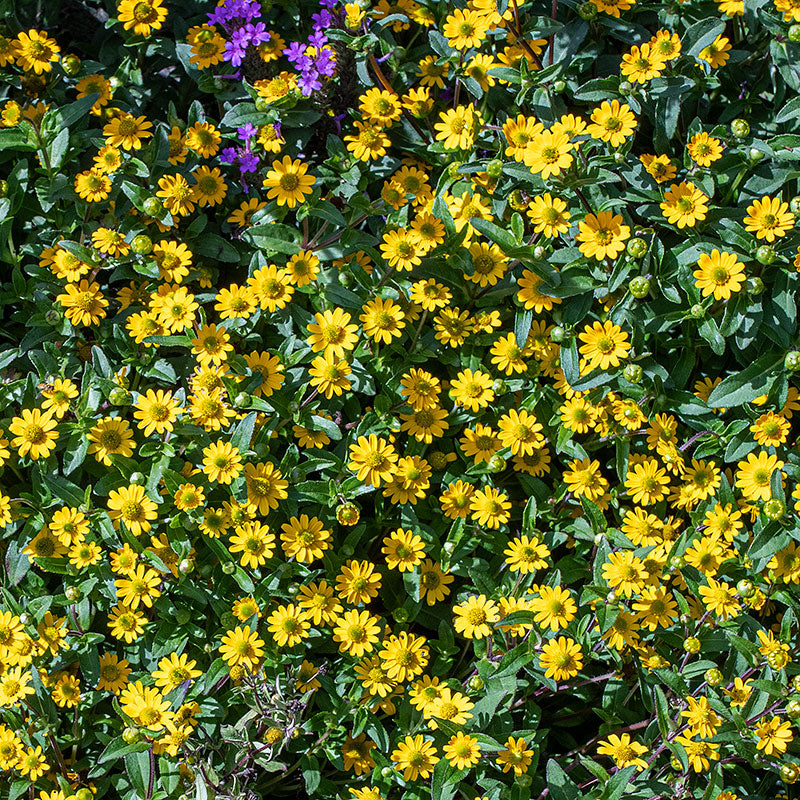The image features a dense cluster of small yellow flowers, likely daisies, with vibrant yellow petals radiating from a greenish-yellow center. Scattered among them, primarily in the upper left, are several small purple flowers that add a contrasting touch. The flowers are at different stages of bloom, with some fully open and others still in unopened or partially opened bud form. The shiny green leaves, reflecting light and interspersed among the flowers, create a lush backdrop, while deeper shadows between the foliage hint at the depths of the plant growth. The bird's eye view allows a detailed look at the flower heads, showcasing their close arrangement and the mix of flower stages within this verdant and colorful scene.